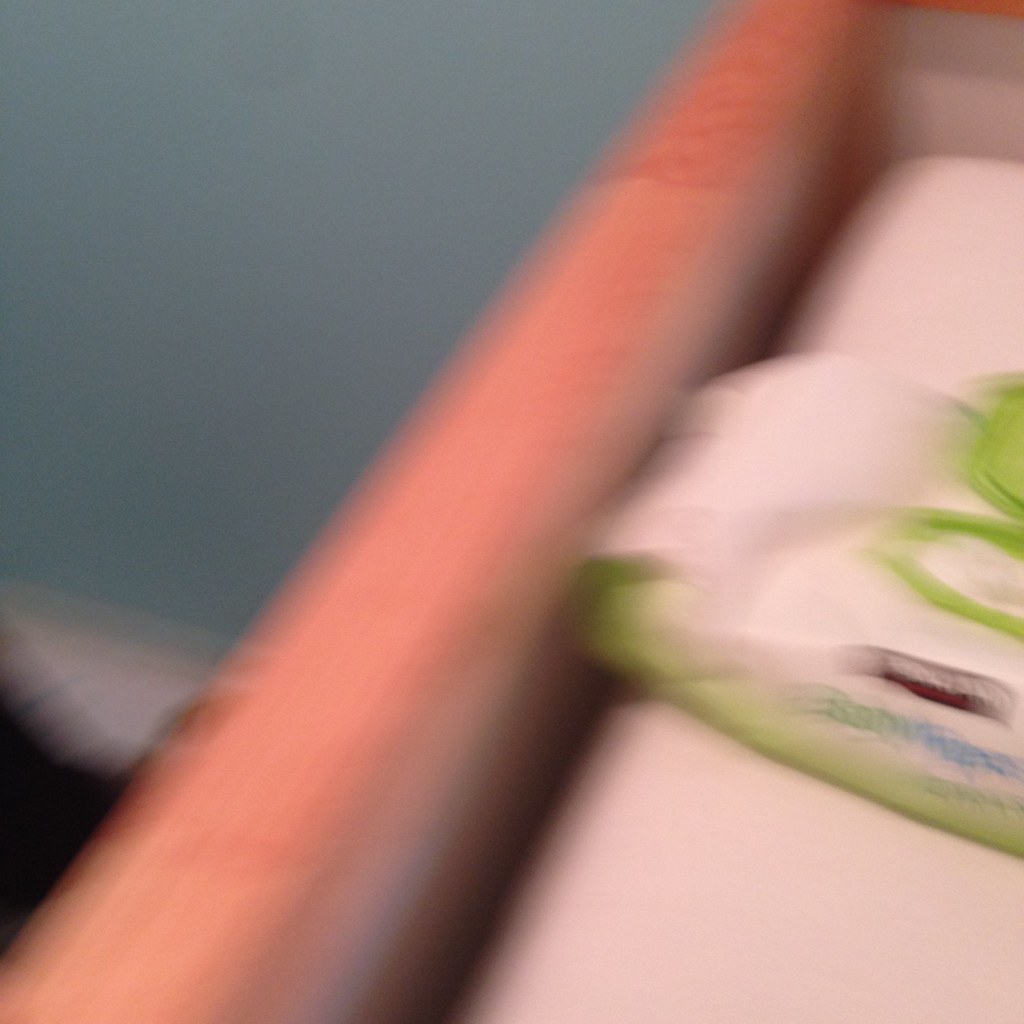The photo is an indoor digital image capturing the upper left to roughly three-fourths of the way across to the right, and about three-fourths of the way down on the left side, featuring a fairly nice blue background. The rest of the photo on the right side is predominantly black. However, emerging from the bottom left corner, extending to the center, is a light tan-colored, cylindrical object. Upon closer inspection, it becomes evident that the object is part of a baby changing table, crafted from a nice white wood. 

On top of the changing table, there is a white mattress designed for a baby or toddler. Positioned in the middle of the mattress is a package of baby wipes. The package is primarily white, with a green lid on the right side that is popped open, revealing the white baby wipes inside. The front of the package features the green accent at the top and bottom, with a black square displaying the brand name "Kirkland" in white print. Beneath "Kirkland," the word "Signature" is written in red cursive. Additional text on the package confirms they are baby wipes, with "Baby" written in green and "Wipes" in blue.